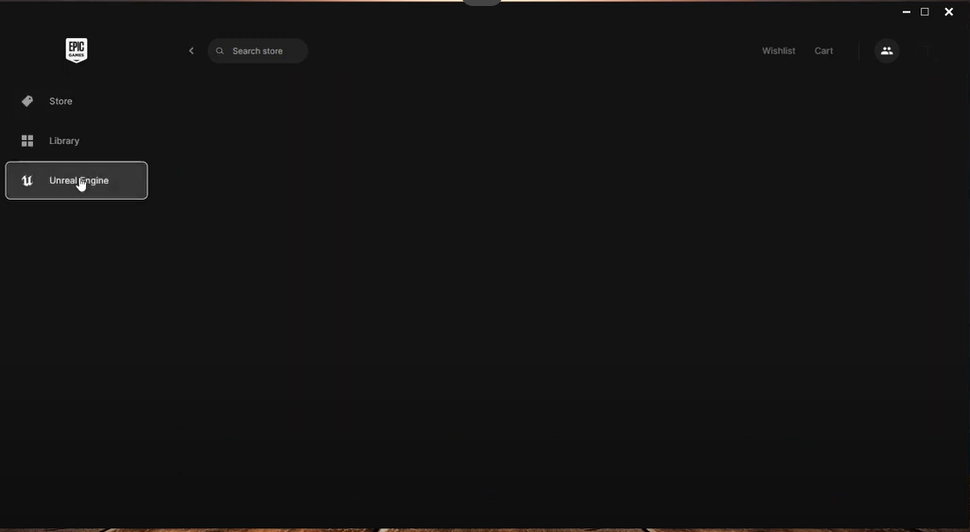The image appears to be a screen capture of a software interface, likely from a computer screen. The background is predominantly black, adorned with a combination of white and gray text and icons. In the top-left corner, there is a series of control icons, including a white minimize symbol, a gray square that represents the maximize or restore function, and a white 'X' for closing the window.

On the right side of the image, the text "Epic" is clearly visible, accompanied by a white shield icon. The font beneath "Epic" is too small to decipher precisely. Below this section, there is a mini-menu featuring three categories: "Store," indicated by a price tag icon in gray, "Library," represented by four small squares, and "Unreal Engine," denoted by a "U" icon. A white mouse cursor, in the form of a hand, hovers around the letter 'E' in "Unreal Engine."

To the right, there is a navigational back arrow and a search box labeled "search store," including a magnifying glass icon. The bottom portion of the screen displays a partial view of what appears to be computer wallpaper, showing only a small, unidentifiable brown object, hinting at more detail behind the black interface.

Just below the minimize, maximize, and close icons, gray text reads "Wishlist" and "Cart," along with a circular icon depicting two white cartoonish figures symbolizing user interaction. The image overall serves to capture the detailed layout and various elements of a user interface, potentially from the Epic Games Launcher or a similar application.